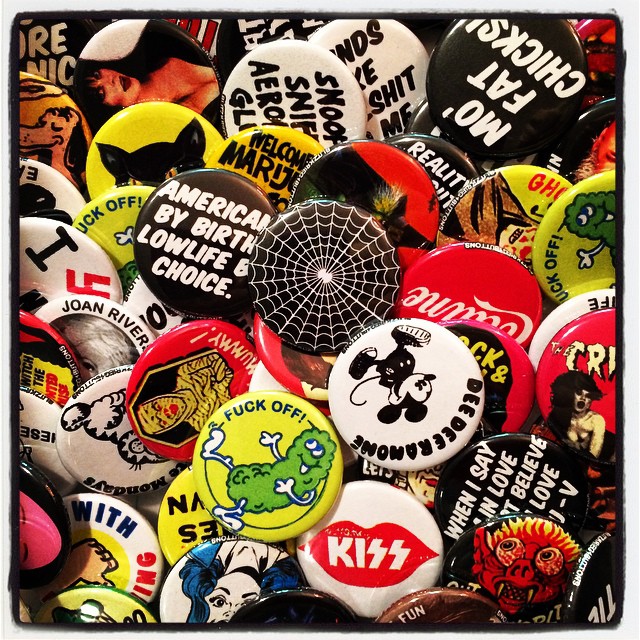This is a square photograph framed by a black boundary, depicting a chaotic, colorful pile of round buttons, each the same size but featuring a variety of designs, slogans, and characters. The image is filled exclusively with these buttons, eliminating any background or external objects. Among the multitude, a few notable buttons stand out: one features the F word with a little green monster; another showcases Mickey Mouse with D.D. Ramone text on a white background. There's a black button with a spiderweb design, and another black one with white text stating, "American by birth, low life by choice." A button with a Coca-Cola logo is present, along with a colorful portrayal of cartoon figures. There's a punk rock vibe punctuated by a button displaying "Kiss" for the band, and another with Elvira's image. An array of vibrant buttons—red, yellow, white, black—include whimsical designs like a poop emoji saying "Fuck Off," a button with Joan Rivers' image, a cat, and a character with an upside-down face. Also included is a button featuring "MoFatChicks" and another yellow one with a humanized pickle saying "Fuck Off." Some buttons are partially obscured due to the overlapping arrangement, but their collective vibrancy and diversity create an engaging, slightly rebellious tapestry.